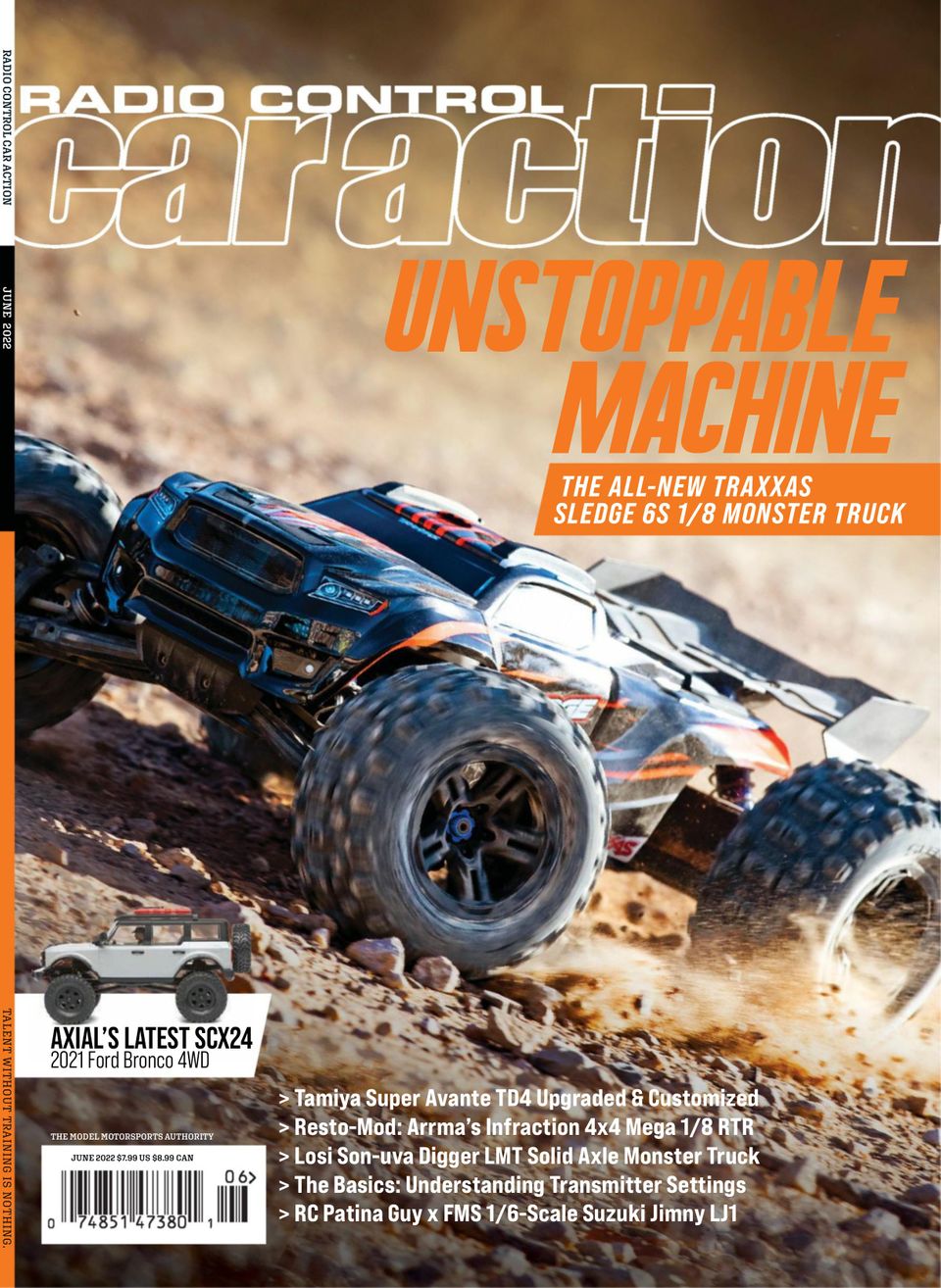On the front cover of a hobbyist magazine titled "Radio Control Car Action," an eye-catching visual of a powerful radio-controlled car commands the layout. The image, which measures approximately five inches high and four inches wide, showcases a black remote-controlled car with a streamlined body and large studded tires climbing a rocky slope. The car is positioned dynamically, moving from the bottom right toward the upper left, emphasizing its off-road capabilities.

At the top of the frame, the magazine's title "Radio Control Car Action" is prominently displayed in white print with a black outline, set against a white background. Just below, an orange headline in uppercase italic font reads "Unstoppable Machine," highlighting the featured article. Beneath this, an orange banner with smaller white text announces "The All-New Traxxas SLEDGE 6S 1/8th Monster Truck."

The cover also provides additional content details in smaller fonts. In the lower left corner, a white rectangle contains a black universal pricing code, adjacent to an image of a white truck with borders, identified as Axial's latest SCX24 2021 Ford Bronco 4WD. To the right of the barcode, a list of other articles is visible in white print against a black background, including pieces on the Tamiya Super Avante TD4, Resto-Mod Armas Infraction 4x4 Mega 1/8 RTR, Losey Sun UVA Digger LMT, understanding transmitter settings, and the RC Patina Guy X FMS 1/6 scale Suzuki Jimmy LJ1.

Furthermore, a thin border about an eighth of an inch wide runs down the left-hand side, with text in various prints and colors, including a black-and-white reminder of the edition being June 2012 and an inspiring quote at the bottom: "Talent Without Training Is Nothing."